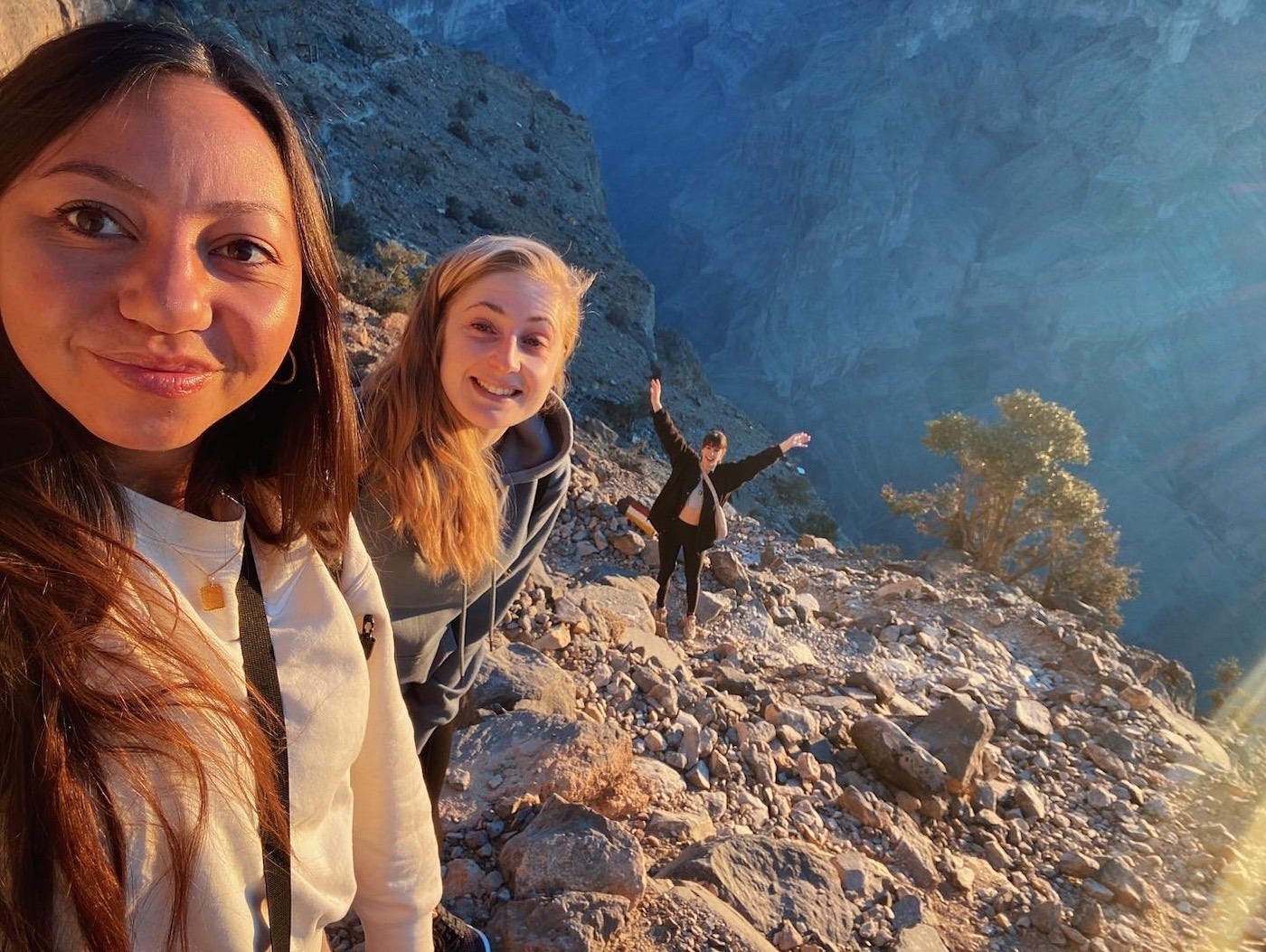This photograph captures three women, evidently hiking and adventuring on a steep, rocky mountain ledge overlooking a canyon. The scene is set in a sunny outdoor environment, dominated by earthy tones of brown and gray rocks, with a distant blue tint and the warm amber glow of sunlight. 

In the forefront on the left, the woman taking the selfie has light brown skin, long straight dark hair, and is wearing a white shirt. She is smiling brightly at the camera. Just behind her stands a second woman with long blonde hair, also smiling warmly. She is dressed in a gray sweatshirt. Further back, near the edge of the cliff, a third woman stands triumphantly, her arms raised high—a joyful wave. Clad in black attire with a purse slung across her body, she exudes excitement and adventure. To the right side of the image, there is a single small green tree amidst the rocky terrain, adding a touch of vibrant life to the rugged landscape.